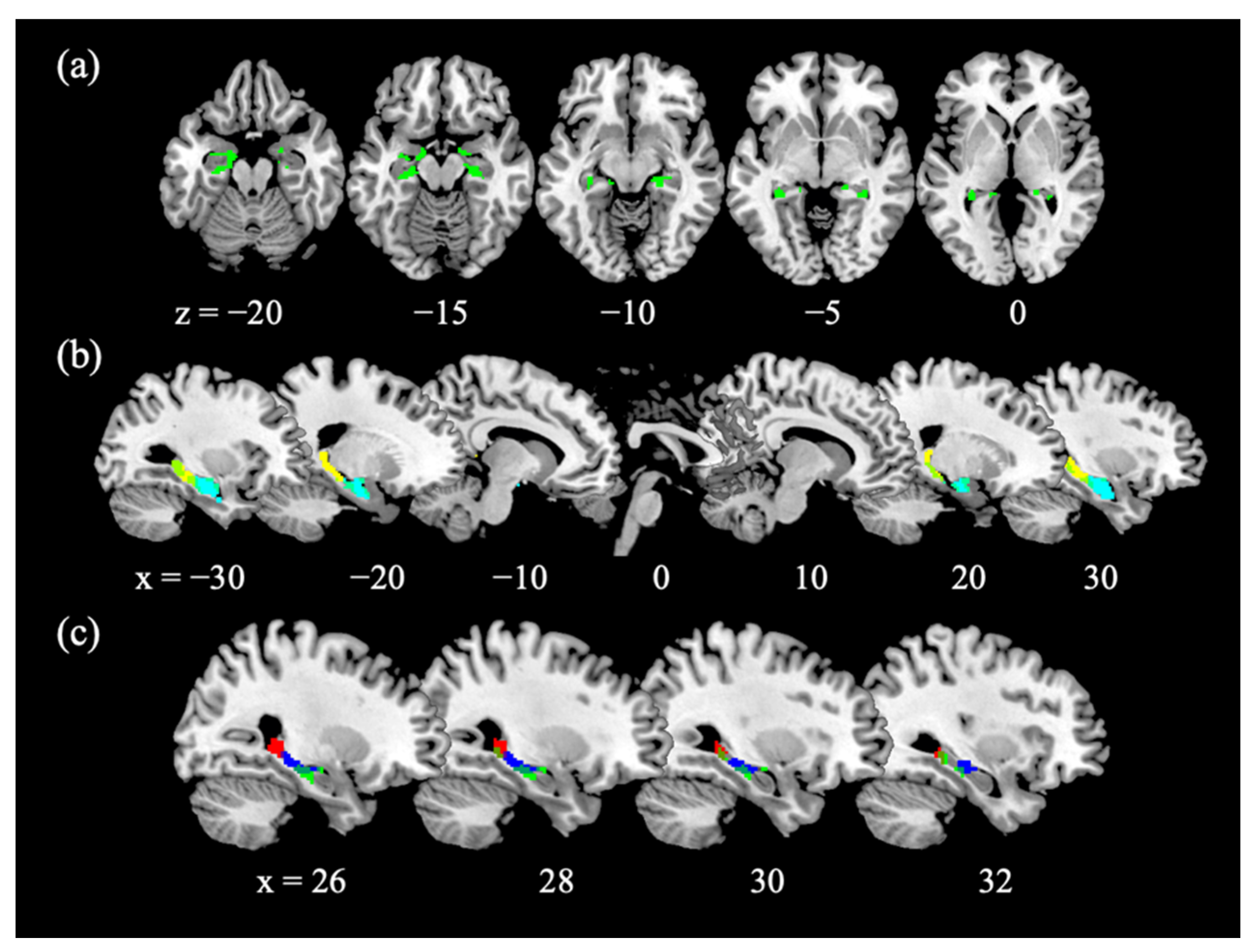This medical image presents a segmented view of a cat's brain, divided into three horizontal sections labeled (A), (B), and (C) in white font at the upper left-hand corners of the respective sections. 

Segment (A) displays a horizontal cross-section of the brain, characterized by a predominantly gray structure with highlights of green on the top. The section includes markings for Z-axis values at intervals of -20, -15, -10, -5, and 0. 

In segment (B), the image shifts to a different representation, marked by X-axis values ranging from -30 to 30 at intervals of 10. This section features the central part of the brain, illustrating areas in green, yellow, and light blue hues.

Segment (C) provides four distinct images, each annotated with specific X-axis values of 26, 28, 30, and 32. These images capture the central regions of the brain with varying colors, including red, blue, green, and lime green.

Overall, the image provides detailed color-coded representations to highlight specific areas of interest within the cat’s brain across different sections and axes.